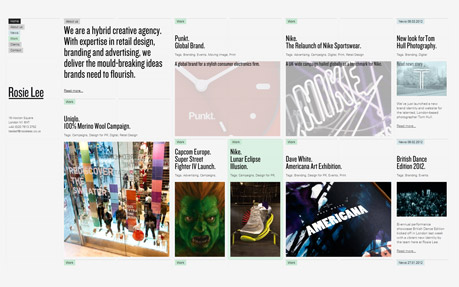The image features Rosie Lee on the left-hand side, nearly center-aligned within the frame. Beneath her name, "Rosie Lee," a brief blurb of text is visible. Approximately four spaces above Rosie Lee's name, there are six words stacked vertically, one above the other.

To the right of Rosie Lee, the main section of the webpage is displayed. This section is organized into two rows. The top row includes the text: "We are a hybrid creative agency with expertise in retail design, brand, and advertising. We deliver the mold-breaking ideas brands need to flourish."

On the left side of this text, there is a prominent punk icon. Below this icon, there is a distinctive block design which appears to be affiliated with Nike.